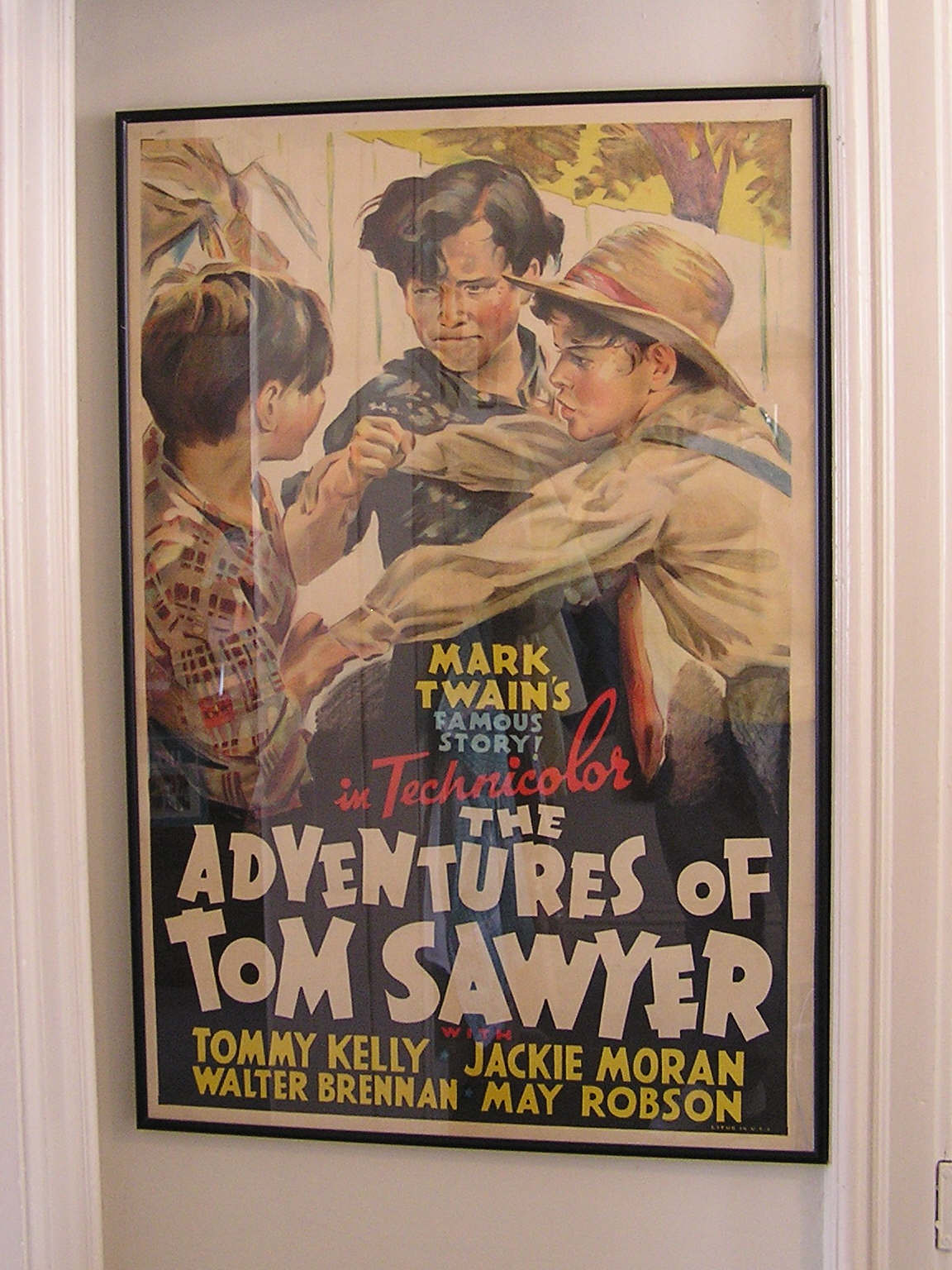The photograph captures a framed movie poster displayed on a gray strip of wall between two white door frames, with the right door slightly open, revealing its hinges. The poster, encased in a sleek black frame with a clear cover, features a watercolor illustration depicting a scene from "The Adventures of Tom Sawyer." The illustration shows three Caucasian boys who appear to be in a confrontation near a white fence, beneath a yellow sky with distant trees. 

The leftmost boy, seen in profile, wears a straw hat with a red band, a white shirt, and denim overalls. The central boy, standing behind the first, has dark hair and looks down wearing a black shirt. The rightmost boy, who faces away from the viewer, has short dark hair and wears a red and white plaid shirt. 

Text details overlay the image: the top announces "Mark Twain's Famous Story," with "Mark Twain" in yellow, "Famous Story" in light blue, and "in Technicolor" in red. Below the illustration, the title "The Adventures of Tom Sawyer" is prominently displayed in bold white print. Beneath the title, the actors' names are listed: Tommy Kelly, Jackie Moran, Walter Brennan, and Mae Robson.